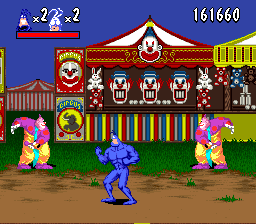A nostalgic screenshot from a vintage NES-style video game captures a lively carnival scene. The small image centers on two clowns standing on a grassy area—one on the left and one on the right. Between them, on a dirt path, stands the main character, a blue-clad figure with a white face. The backdrop features a vibrant carnival game with a trio of clowns flanked by two bunnies on either side, and a colorful rainbow pattern below. Topping off this whimsical setup is a red and white circus tent, complete with a central clown figure, enhancing the festive atmosphere.